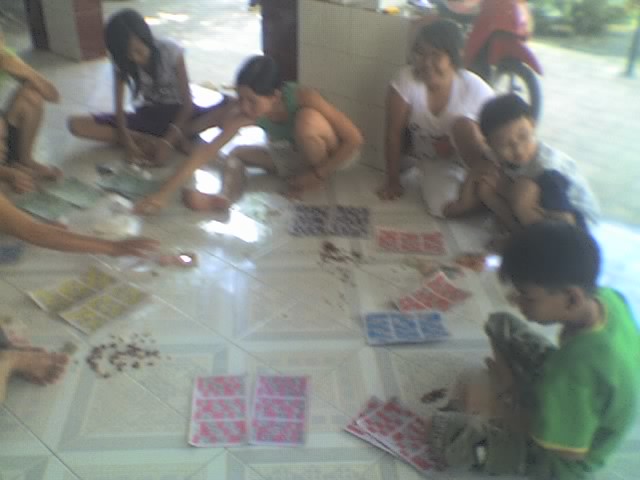The image captures a somewhat blurred scene of children and teachers engaged in a game, possibly resembling bingo, on a patterned linoleum floor. The floor features a subtle mix of light peach and light gray hues. The photograph is taken from a distance, making it challenging to discern the details of the game. Participants, consisting of three females and three boys, hold two pieces of paper each, which appear to have blocked sections in various colors such as red, pink, yellow, blue, purple, and green, often paired with gray. Scattered around them are small, indistinct items associated with the game. A scooter is visible in the background. The setting suggests an Asian country, inferred from the participants' facial features, and the location seems to offer a transition between indoor and outdoor spaces.